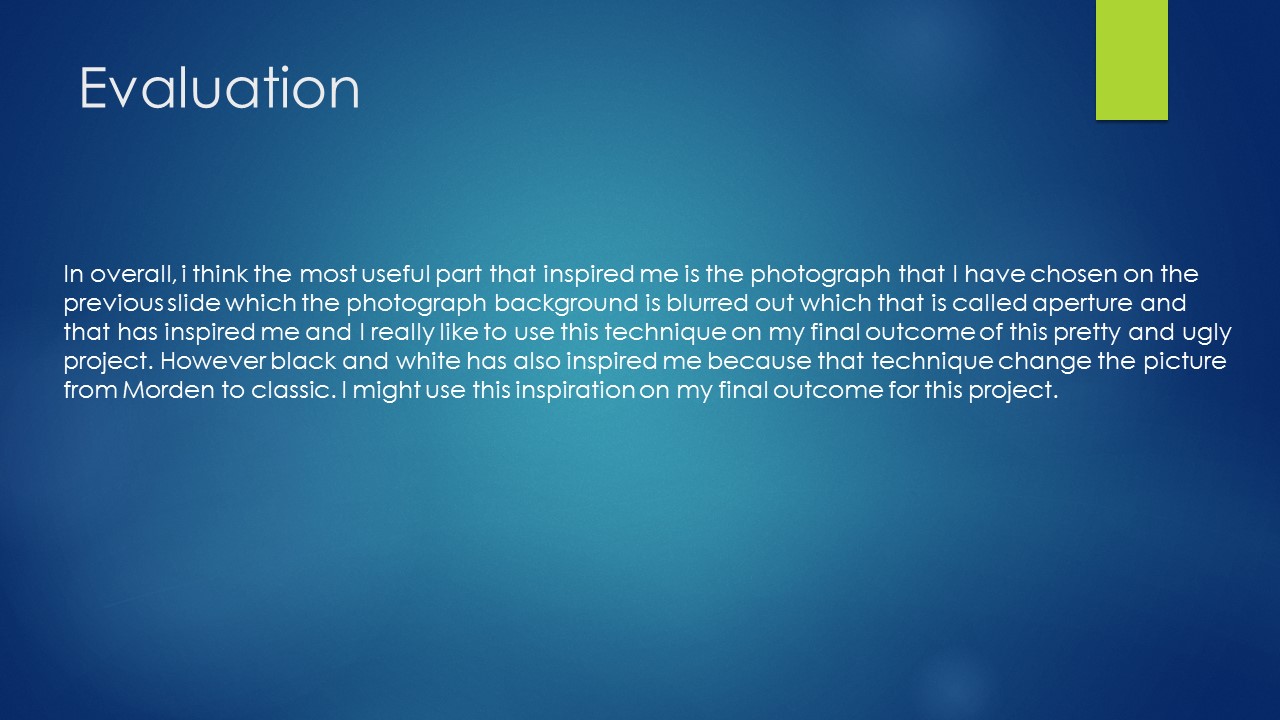The image appears to be a presentation slide with a bluish-white gradient background that transitions from a light grayish-cyan in the center to a darker blue at the edges. At the top of the slide, in bold white text, is the word "EVALUATION." On the upper right-hand side, there's a small lime green bar, possibly indicating a page number. Below the title, a paragraph in white text discusses the inspiration derived from a photograph on a previous slide, particularly appreciating the blurred background effect known as aperture. This technique is favored for its potential use in a "pretty and ugly" project. Additionally, the speaker finds the black-and-white technique transformative, changing the picture's feel from modern to classic, which they also consider incorporating into their final project outcome.